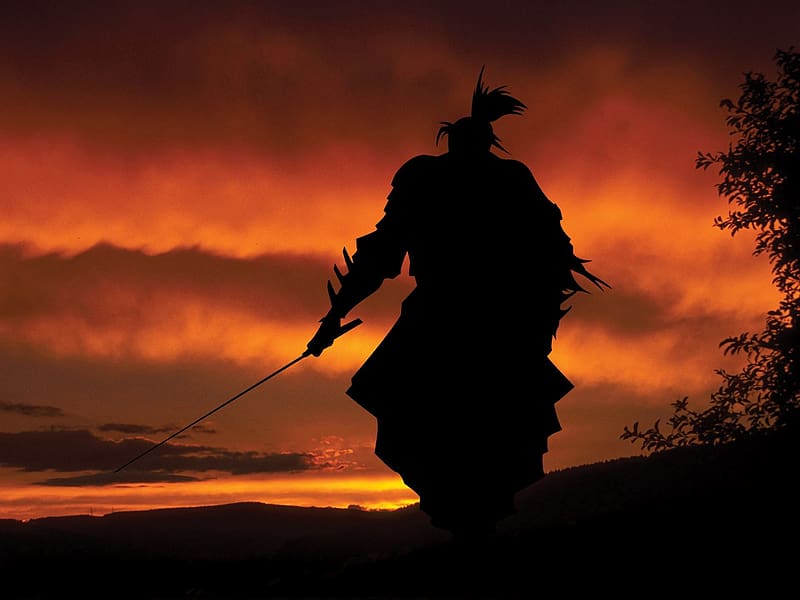The image captures a striking scene that seems to be a blend of both photo-realism and illustration, depicting a sunset bathed in intense hues of orange, red, and yellow, evoking the sense of a sky on fire. Dominating the frame is a silhouetted figure of a samurai, back turned to the viewer, standing on a dark, possibly elevated ground. He wears a long, dark garment adorned with protruding elements, possibly armor, and a helmet topped with black feathers. The samurai holds a long, thin katana in his left hand, pointed downward. To the right, the dark silhouettes of bushes or trees frame the scene, adding depth to the fiery, wavy clouds and lightening horizon at the bottom. The image effectively uses the interplay of bright, blazing sky and dark shadows to create a powerful and dramatic atmosphere.